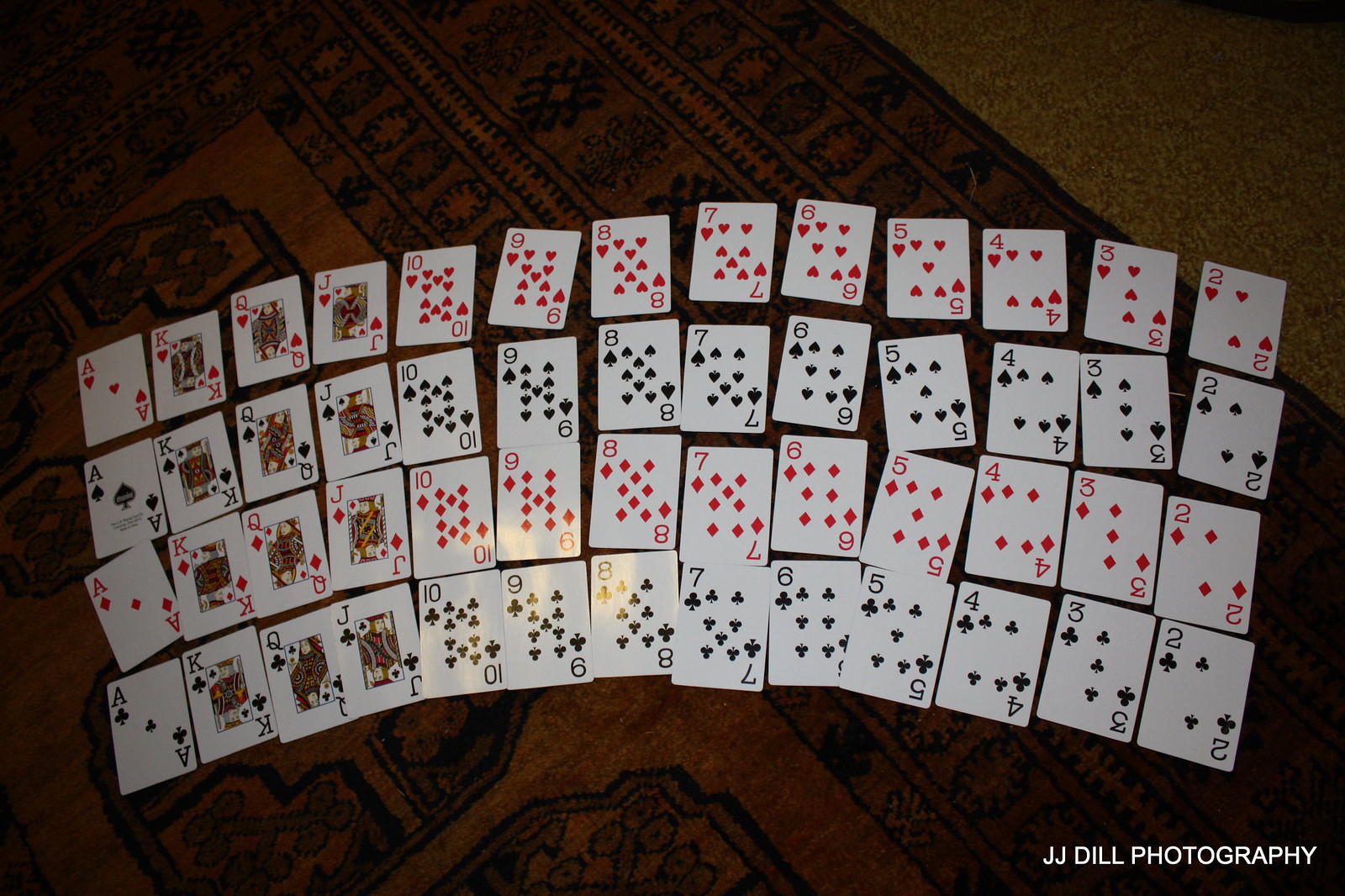In the image, a deck of cards is meticulously laid out on a table in a landscape orientation. The cards are arranged in four rows, each representing one of the four suits: hearts, spades, diamonds, and clubs. Each row consists of 13 columns, starting with an Ace and followed sequentially by the King, Queen, Jack, 10, 9, 8, 7, 6, 5, 4, 3, and 2. The first row features the suit of hearts, the second row is dedicated to spades, the third row to diamonds, and the fourth row to clubs. The table under the cards has a subtle, dark design that is difficult to discern. A light source positioned above casts a reflection on the lower two rows of cards, specifically illuminating the 10, 9, and 8 cards.